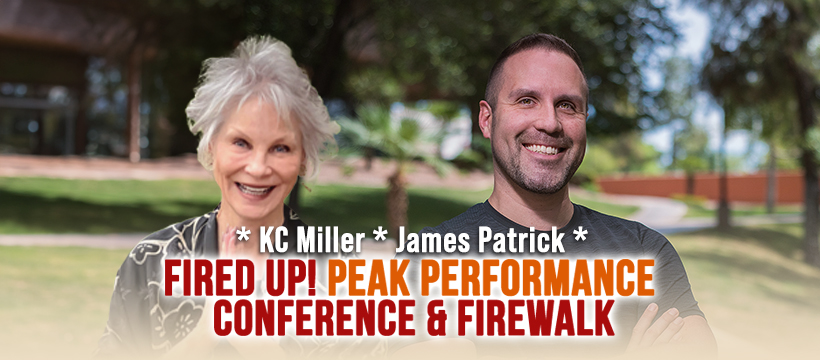The image is an advertisement for a conference and firewalk event featuring Casey Miller and James Patrick. They are pictured standing next to each other in an outdoor park-like setting with green grass, trees, and a blurry background that includes a reddish-brown fence to the right and a building to the left. Casey Miller, an older woman with whitish-blonde hair, is on the left. She has very thin eyebrows and a wide nose, and is smiling at the camera, raising her hands in front of her. She is wearing a gray and white shirt. On the right stands James Patrick, a man with short, dark hair, especially short on the sides, and a stubbly beard. He is also smiling at the camera with his arms crossed, dressed in a gray t-shirt. The promotional text in the middle of the photo reads "FIRED UP! Peak Performance" in red and orange, and below, "CONFERENCE & FIREWALK" in red all caps.